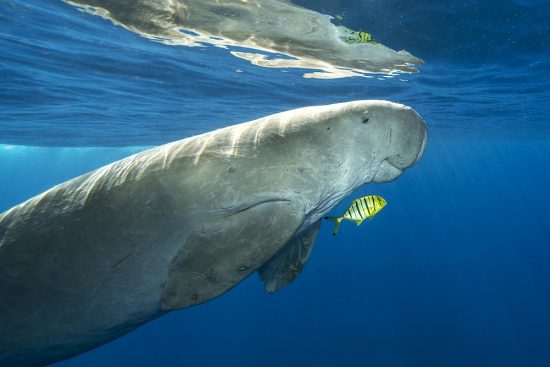This detailed underwater photograph features a large, gray manatee, which is the central focus of the image. The manatee is swimming near the surface in clear, very blue water, with its body emerging from the bottom left-hand corner and moving towards the upper right-hand corner of the frame. The water's surface creates a reflection of the manatee above it, adding a sense of depth to the scene. The manatee’s body is textured with lighter shades underneath and striping on top, likely from the light reflecting off the water. Notably, the manatee has what appears to be a pleasant smile on its face, enhanced by its tiny eye and the wrinkles below its chin. Its flippers are tucked back, resembling those of a turtle. Accompanying the manatee is a small, distinctive fish positioned just below its neck. This fish is characterized by its yellow body with black and white stripes and is swimming in parallel with the manatee towards the same direction. Both creatures are illuminated by the gentle light filtering through the water, creating a serene and harmonious underwater scene.